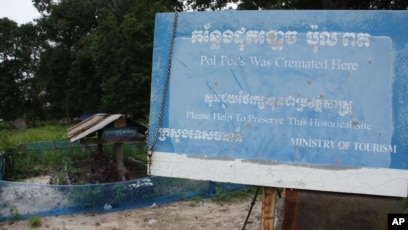The image depicts a potentially historic site marked by a light blue sign on the right-hand side, partially cutting into the middle of the image. The sign is written in both Khmer and English, indicating that Pol Pot, the infamous Cambodian dictator, was cremated at this location. The English text on the sign reads, "Whole pies was cremated here," followed by, "Please help to preserve this historical site," with a reference to the Ministry of Tourism. The photo appears to be of low quality and slightly blurry, possibly old, with an "AP" watermark in the bottom right corner, suggesting it was sourced from the Associated Press. The sign is set within an outdoor area featuring trees, grass, and a concrete section with a small garden. A structure with a small brown roof, potentially a memorial or well, is visible in the background, enhancing the solemn atmosphere of the site.